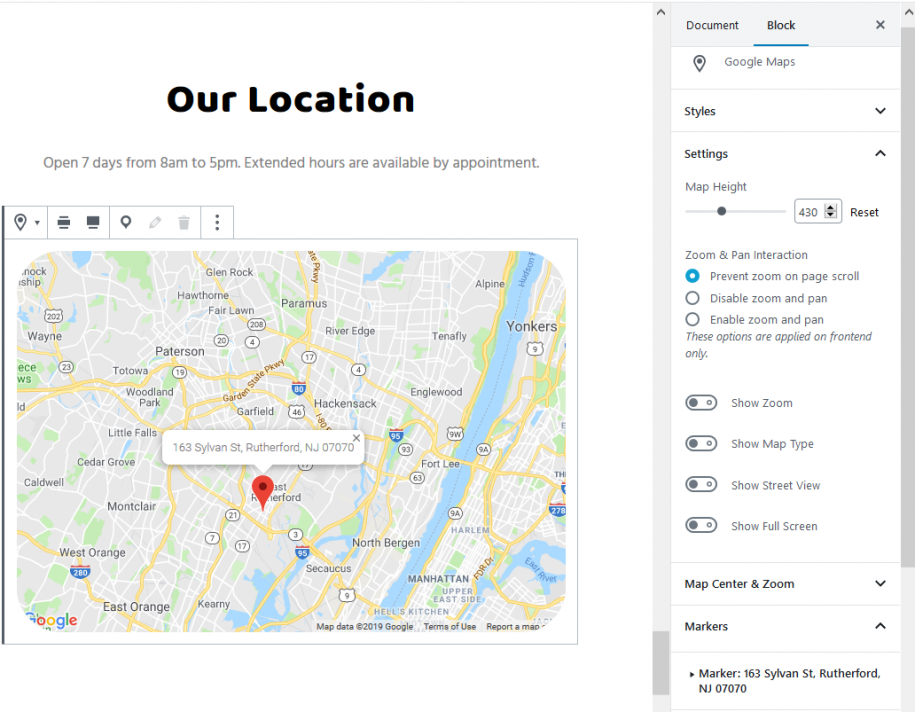This is a screenshot of a web page featuring a mix of layout elements and settings options, likely related to Google Maps. The left side of the page has a white background with black text that reads "Our Location." Below this title, it states, "Open seven days from 8 a.m. to 5 p.m. Extended hours are available by appointment," which is displayed in gray text. Beneath this information, there's a map of New Jersey marked with a red arrow pointing to 163 Sylvan Street, Rutherford, New Jersey, 07070.

On the right side of the screenshot, settings options are visible. At the top of the settings panel, a gray bar contains the options "Document" or "Block," with "Block" being selected. The section below this bar includes various settings under titles like "Google Maps," "Styles," "Settings," "Map Height," "Zoom and Pan Interaction," and "Prevent Zoom on Page Scroll," showing that the "Prevent Zoom on Page Scroll" option is selected. Other settings options allow for toggling features such as "Disable Zoom and Pan" and "Enable Zoom and Pan," with the note that these options are applied on the front end only. Additionally, four toggles labeled "Show Zoom," "Show Map Types," "Show Street View," and "Show Full Screen" can be turned on or off.